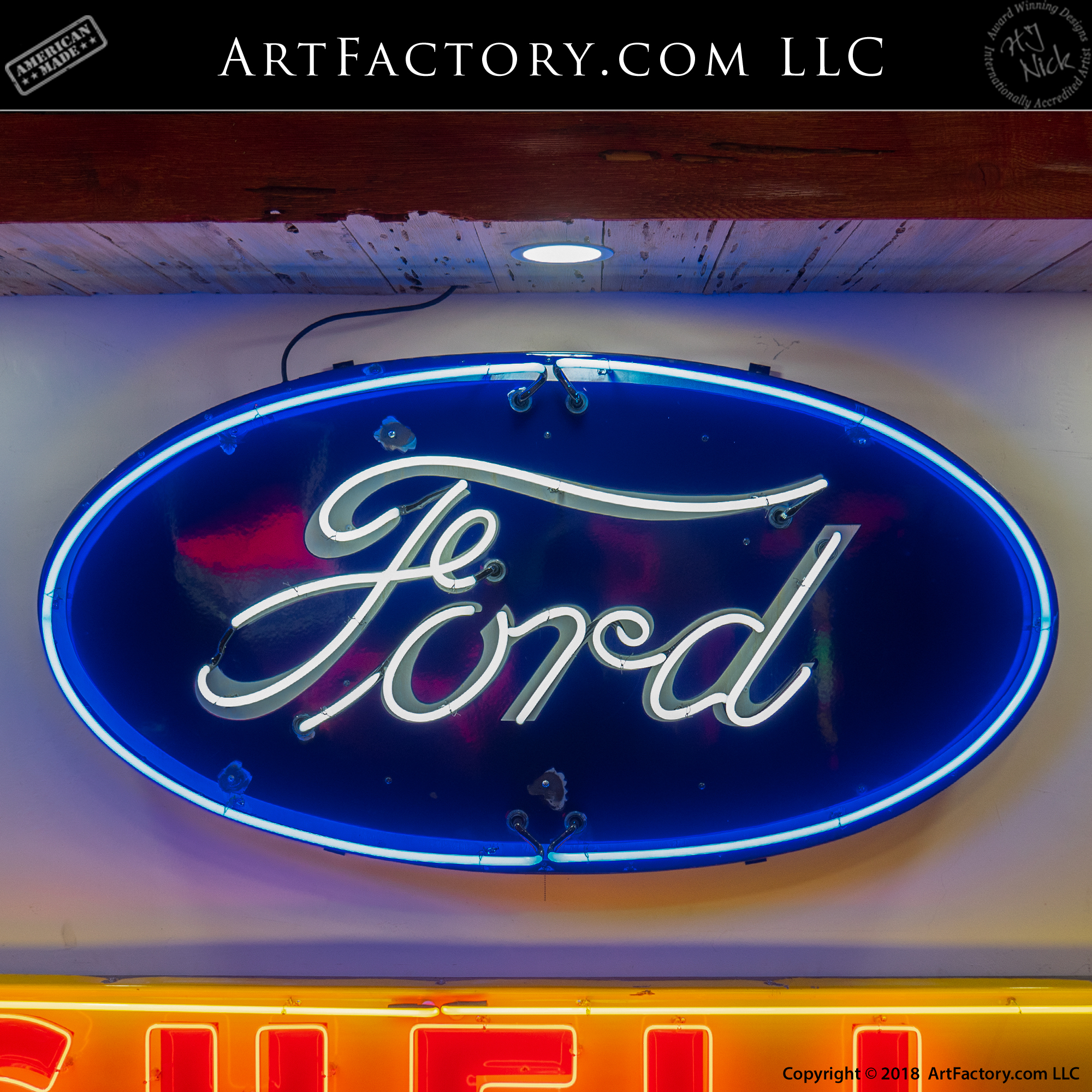This detailed image showcases a prominently large, 3D neon-style Ford logo, prominently featuring a bold, oval-shaped blue background with the iconic white Ford font. The logo is the central focus, suspended on a white wall and accompanied by another partially visible neon light display beneath it, likely reading "Shell". The setting includes a wooden ceiling with a spotlight directly above the logo.

At the top of the image, a black banner with white text reads "American-Made, ArtFactory.com, LLC" on the left, while the right features a watermark of H.J. Nick, noting him as an award-winning, internationally-accredited artist. The circular stamp around H.J. Nick's name enhances the vintage, retro aesthetic of the display. The prevalent colors include shades of blue, white, black, brown, with some red and orange from the underlying partial sign. In the bottom right corner, the text "Copyrights, 2018, ArtFactory.com, LLC" is clearly visible. The overall ambiance melds modernity with a retro touch, epitomizing an artistic representation of iconic automotive branding.